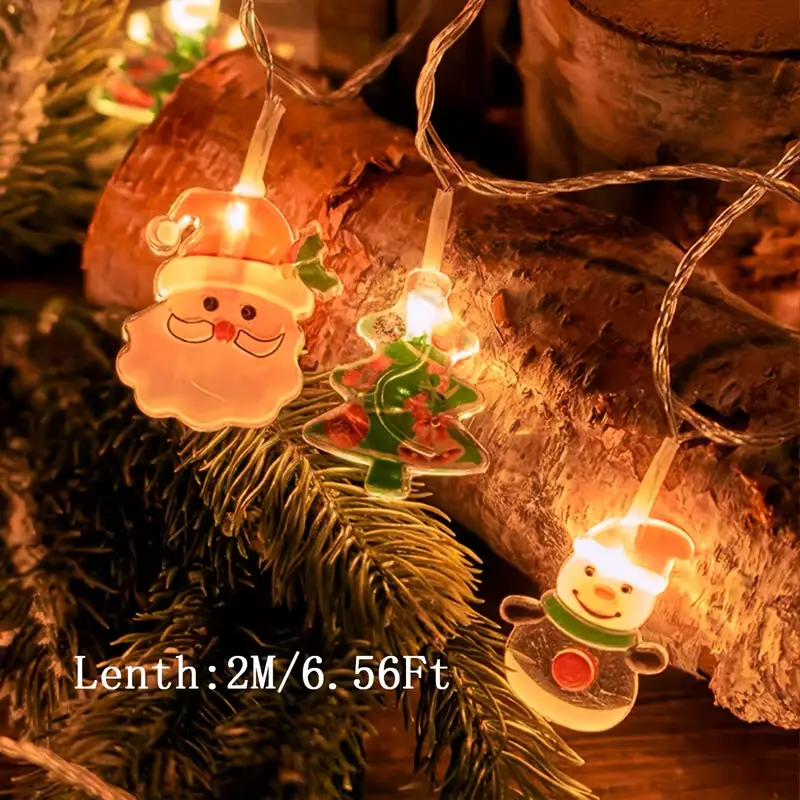In the image, there are three distinct Christmas light decorations arranged on a wooden floor, likely at the base of a Christmas tree. Each decoration is plastic and emits warm white light through small bulbs. To the left, there's a Santa Claus head with a red hat adorned with holly, a voluminous white beard, and small dotted black eyes. In the center, a green Christmas tree light features red accents and candy canes. To the right, a snowman light with small black arms sports a red Santa hat and has a prominent red button on its belly. Notably, there is a watermark at the bottom left corner of the image, which inaccurately spells "length" as "LENTH" and indicates the dimensions as 2 meters (6.56 feet). The decorations are wired together and appear slightly transparent, adding a delicate touch to the festive display.